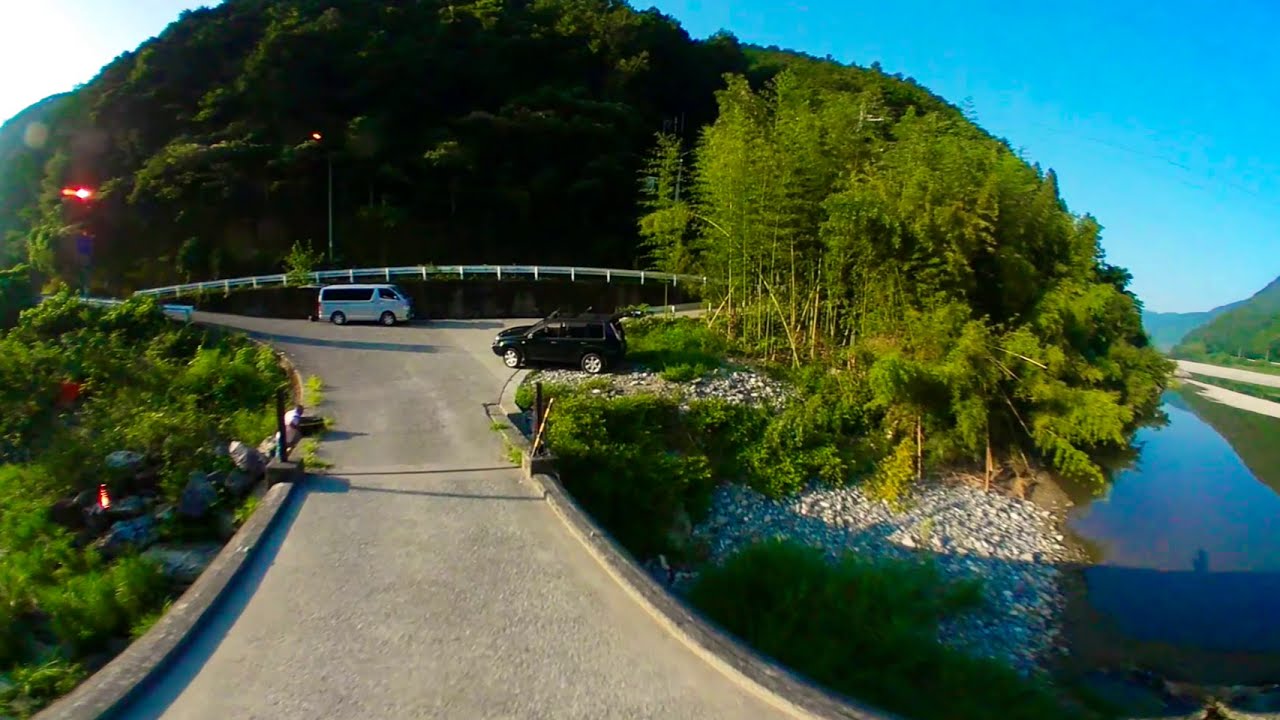The scene captures a serene, outdoor nature setting on a street that leads to a rural park in a mountainous area. On the right, a river or stream flows adjacent to a rocky shore adorned with patches of grass. The dense forest beyond features an intriguing mix of young, thin bamboo stalks resembling reeds and a variety of other very dark green trees, creating a layered canopy. The photograph is taken from a driveway or parking area, with a slight fisheye effect, depicting two parked cars. On the left, a greenery-filled ditch runs parallel to the road, which tees off ahead into a T-junction marked by a white barrier. In the far distance, the landscape transitions into a canyon cutting through the thick forest, encapsulating the untouched beauty of this likely Asian locale. The sun, obscured and off to the left, suggests the photo was taken late in the day.